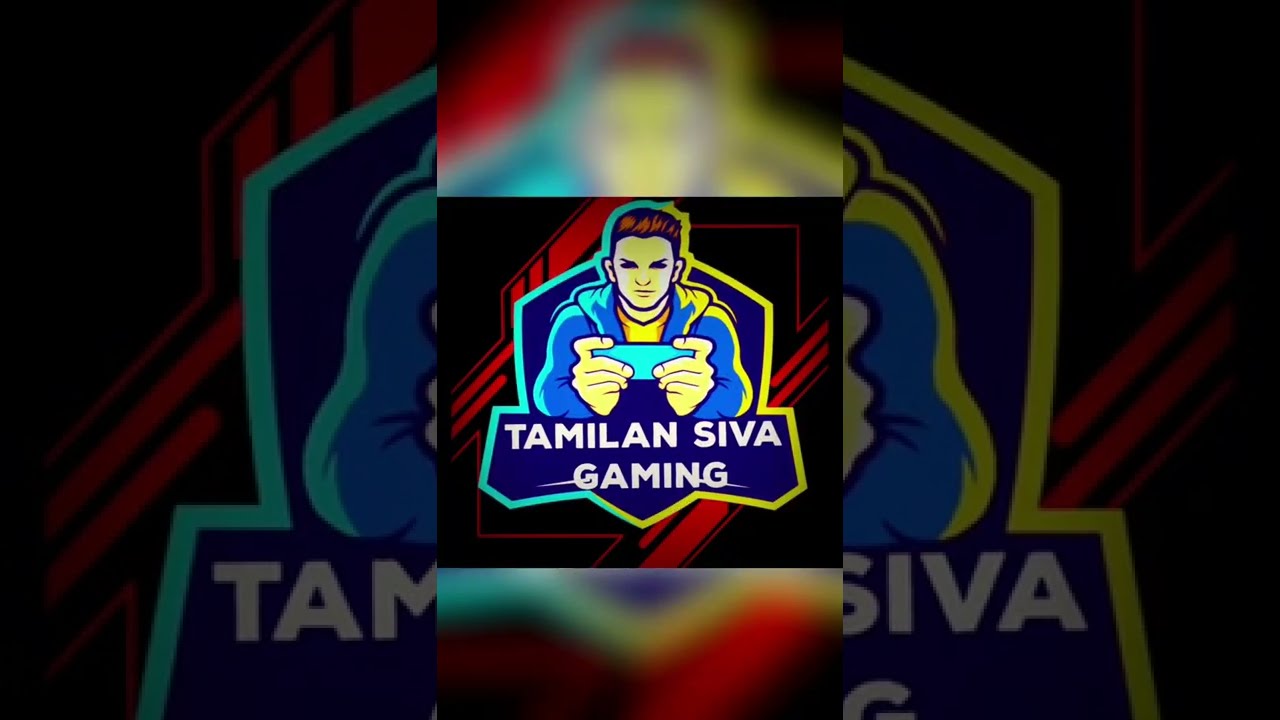The image is a digitally generated graphic of a young man with red hair, wearing a blue hoodie over a yellow t-shirt, holding a light teal-colored game controller in his hands. This main image is centered within a square. Behind it, the same image is repeated in a vertical rectangle that runs top to bottom, slightly blurred to create a diffused light effect. Further in the background, the image is stretched horizontally across the wider screen, appearing faded and darker, providing a subdued backdrop. The central figure, possibly symbolizing a gaming logo or crest, is surrounded by dark blue, yellow, and light teal accents, against a black background with red streaks. Below the main image, white text reads "TAMILAN SEVA GAMING," suggesting it represents a gaming company or brand.